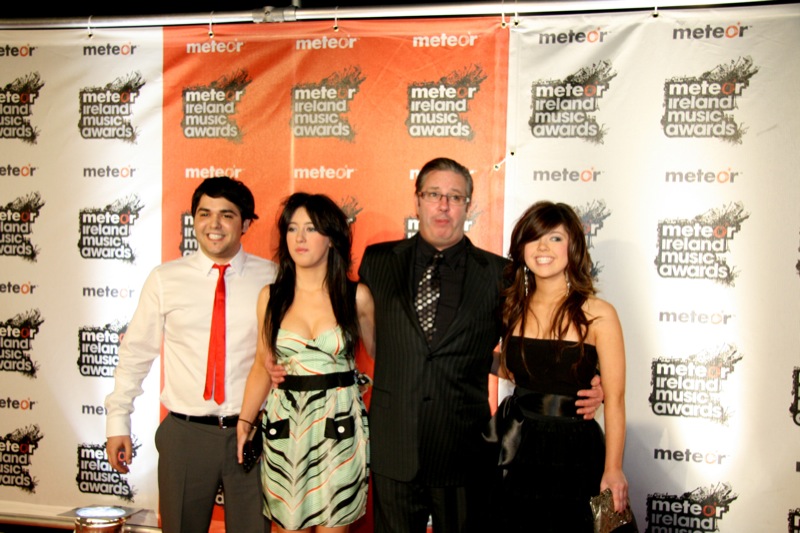In the center of the image, four individuals are standing together, posing for a photograph in front of a backdrop that reads "Meteor Ireland Music Awards." The backdrop consists of a repeating logo with a white section on the sides and an orange section in the center.

On the far left, a young Hispanic man with short black hair parted to the side is dressed in a white long-sleeve, button-up shirt paired with a red tie and gray slacks. Beside him is a fair-skinned woman with long black hair cascading down her chest, dressed in a green dress adorned with a black belt and black pockets. Her dress shows some cleavage, and she is looking slightly to the left.

To her right stands another man, this one wearing a meticulously slicked-back green-white hair, a black suit, and a black-and-white tie. He has glasses on and is gazing to the right, with his arms around the two women beside him. The woman on the far right is dressed in a black dress that ends just above her chest, her shoulder-length dark brown hair partially covering her left eye. She holds a gold-colored purse in her right hand.

The individuals and the colorful backdrop create a vivid and dynamic scene set against the context of the music awards event, with prominent colors being black, white, red, green, silver, and orange. The setting appears to be indoors, illuminated by the event lights.